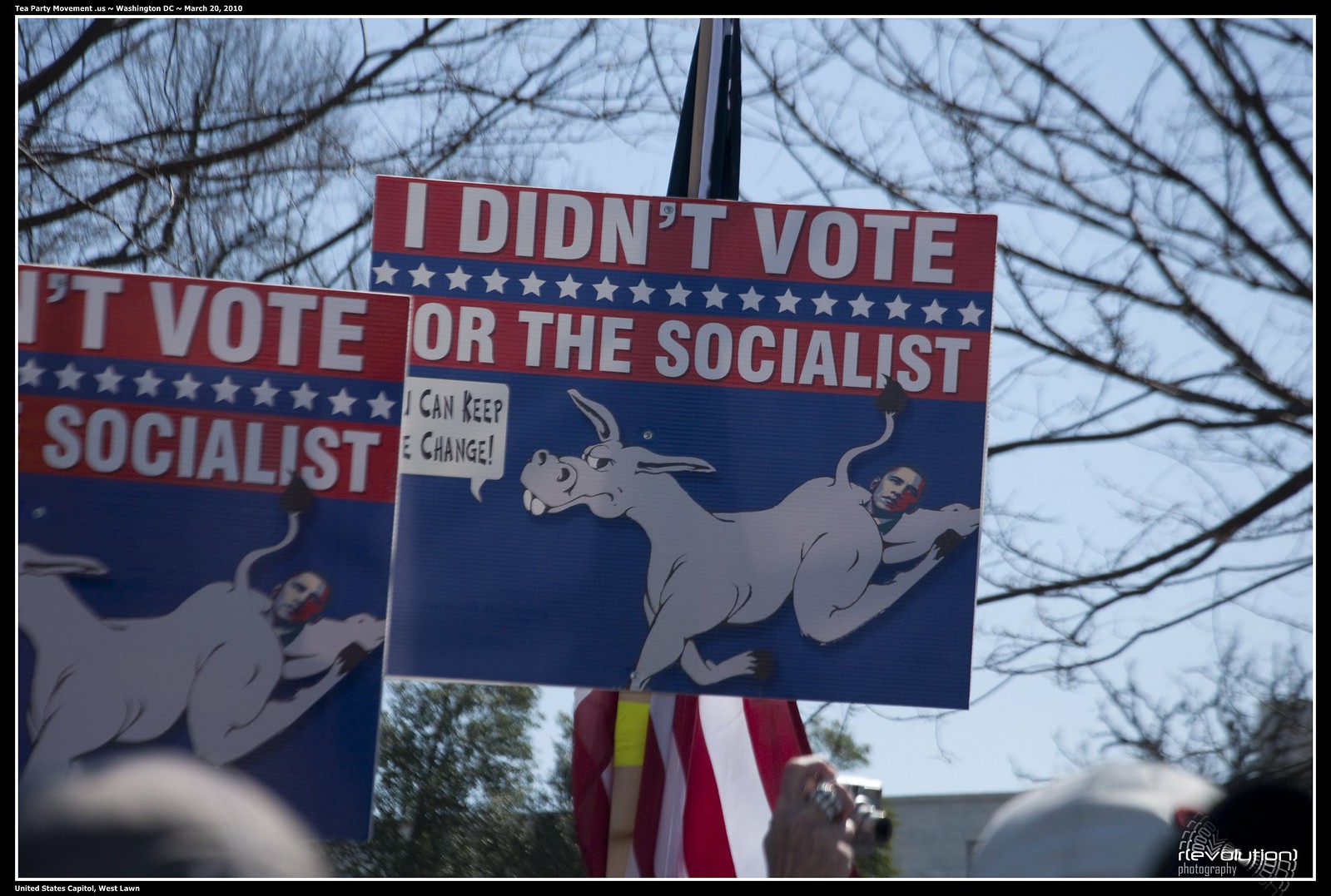This photo, taken outdoors on a clear day, captures a political protest. Prominently featured in the center of the image is a square sign held aloft, emblazoned with the text "I didn't vote for the Socialists" in bold white letters. The sign is rendered in red, white, and blue colors. Below the text, the sign depicts a donkey with an image of Barack Obama's face emerging from its rear end, styled in the iconic blue and red hues reminiscent of his 2008 campaign photos, and accompanied by the phrase, "You can keep the change." To the bottom right of the main sign, another identical sign can be seen held up by another protester. An American flag is visible in the background, hanging calmly due to the still weather. Additionally, the bottom right corner of the image features a logo for Revolution Photography, with the word "revolution" artistically designed to appear as though it's spinning in a circle. The scene is framed by partially visible tree branches and fragments of the sky, while the tops of protester's heads can be faintly seen below the signs.